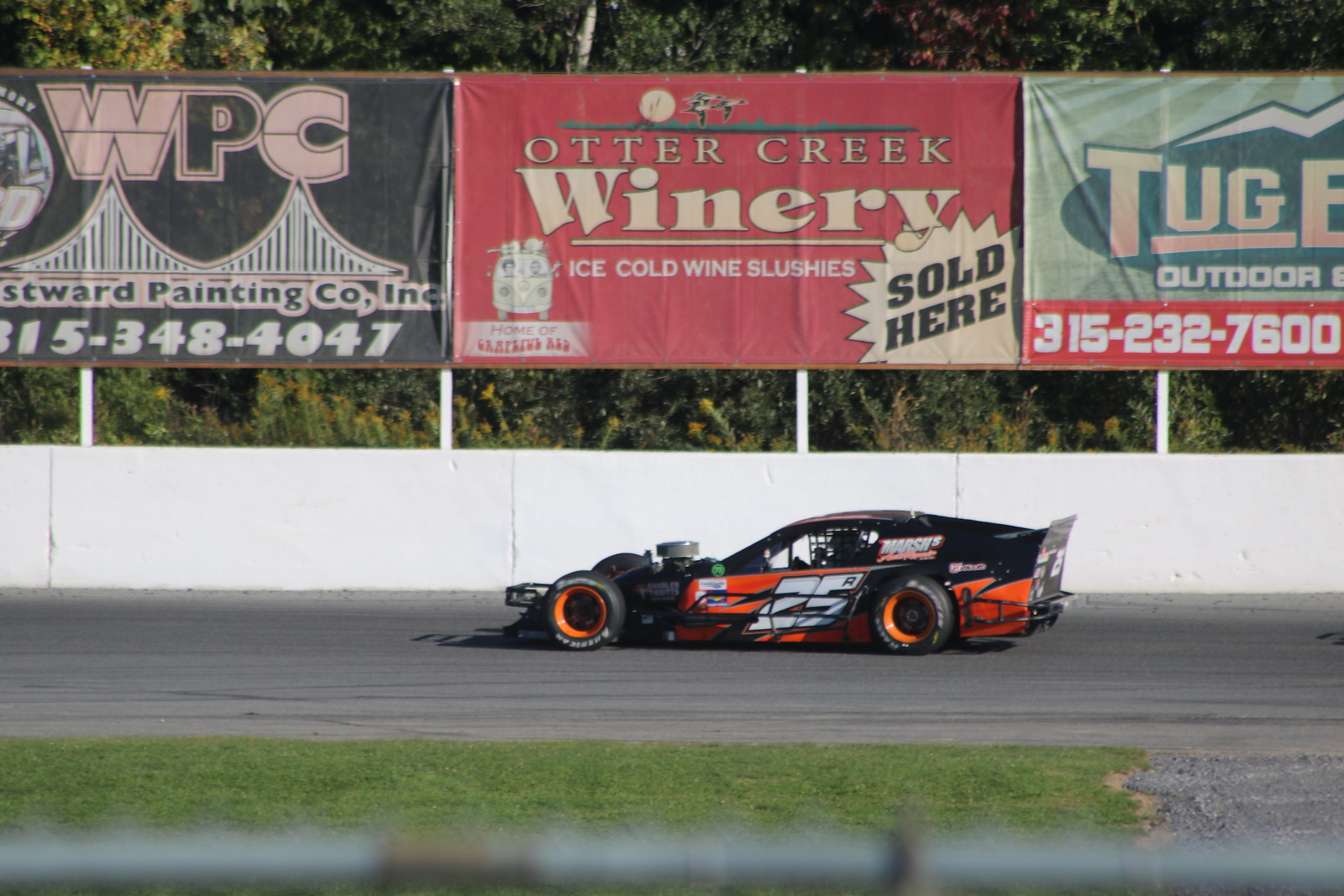This photograph captures an exhilarating moment on the race track featuring a unique racing car. The vehicle, with a closed roof yet open wheels, boasts a front-engine design prominently displaying an air filter atop. This high-performance track car, adorned with striking orange and black colors, is emblazoned with the number 25. Its vivid orange rims immediately catch the eye, contrasting against the darker spokes. The car's rear spoiler adds to its aerodynamic build. It speeds along a racetrack bordered by a white barrier, atop which three advertising signs are visible. In the center of the track, a strip of green grass offers a touch of nature amidst the adrenaline-fueled setting. Clearly designed for racing, this car epitomizes track-only prowess and thrill.